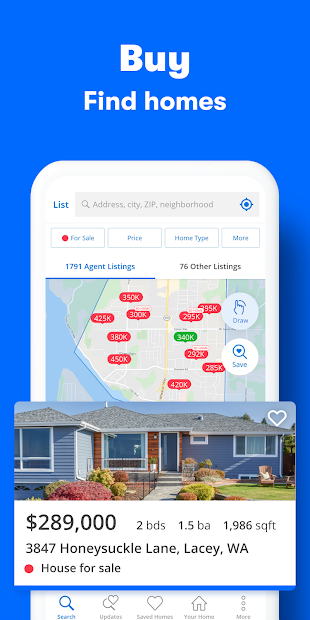The image appears to be an advertisement for a real estate app, showcased against a light blue background. A significant portion of the visual, about a quarter from the bottom, features the outline of a white smartphone. Centrally positioned at the top of the screen, the word "Buy" is displayed in bold white letters, followed by "Find Homes" directly beneath it.

The app interface includes a search section where users can enter an address, city, or zip code. Adjacent to this input field on the right side is a GPS location icon. Below the search options, there are filters for "For Sale," "Price," "Home Type," and "More." Beneath these filters, a map is displayed with various colored dots representing different listings. These dots are primarily red, with one green icon, each labeled with a price.

The map also indicates that there are 1,791 listing agents available and 76 additional listings. In the lower portion, a detailed listing of a specific house is shown. The house is blue with a white heart icon situated at the upper right-hand corner of its image, signifying it as a saved or favorited listing. Below the image, the listing details include the sale status, the number of bedrooms and bathrooms, total square footage, and the complete address. A red dot at the bottom of the listing confirms the house is for sale.